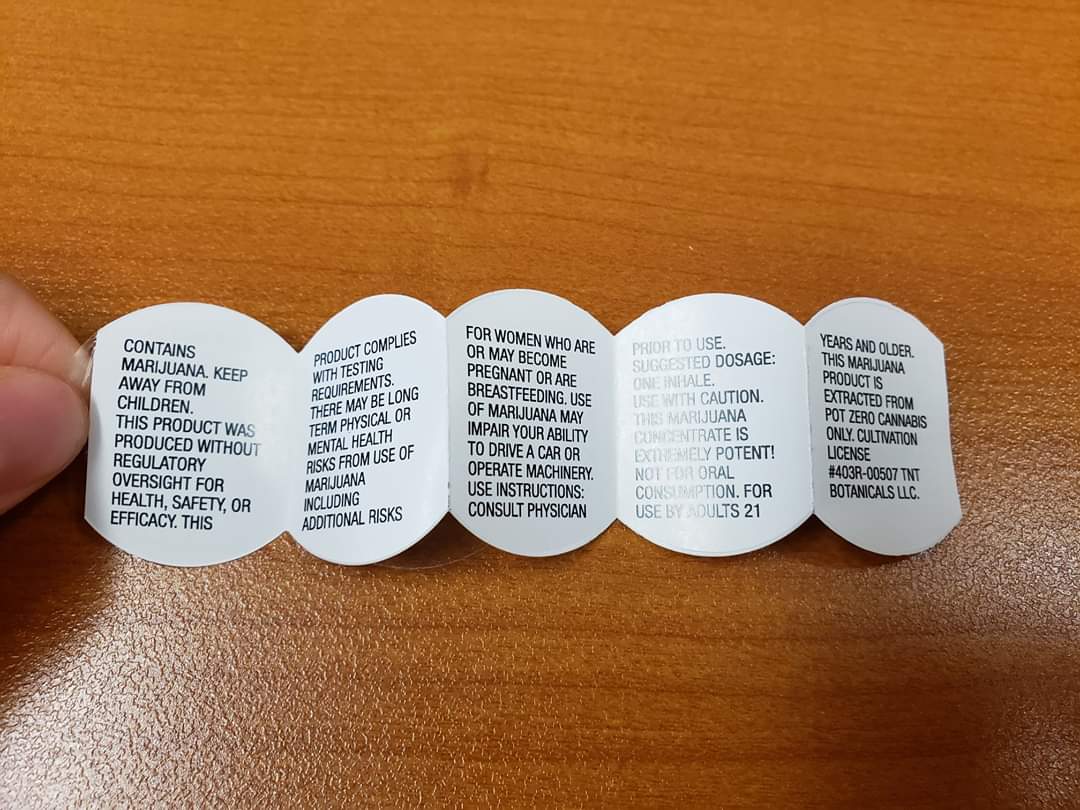The image depicts a white, circular warning tag with one straight edge, lying on a wooden table. The tag is extended like an accordion, revealing multiple warning labels, and is held at one end by a thumb and index finger, with the shadow of the hand visible on the table. The text on the tag reads: "Contains marijuana. Keep away from children. This product was produced without regulatory oversight for health, safety, or efficacy. Product complies with testing requirements. There may be long-term physical or mental health risks from the use of marijuana, including additional risks for women who are or may become pregnant or breastfeeding. Use of marijuana may impair your ability to drive a car or operate machinery. Use instructions: consult your physician prior to use. Suggested dose: one inhale. Use with caution. This marijuana concentrate is extremely potent. Not for oral consumption. For use by adults 21 years and older. This marijuana product is extracted from Pot Zero Cannabis only. Cultivation license number 403 R-00507. TNT Botanicals LLC." The detailed warnings emphasize the product's potential risks and regulatory status, making it clear that it is a marijuana product intended only for adult use.